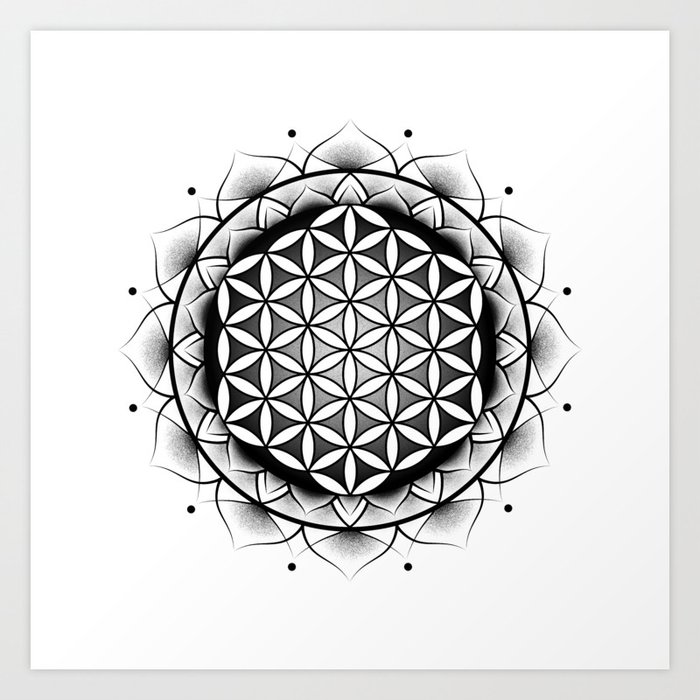This black-and-white image is a highly detailed pencil or computer-generated drawing, presented against a white background and enclosed by a thin gray frame. The drawing centers on a complex, geometric mandala design reminiscent of East Asian art, featuring a "Flower of Life" pattern. The outermost edge of the mandala is defined by translucent white triangular petals, each marked with a black dot at its pointed tip.

Moving inward, the pattern alternates between dark and light areas, creating a shaded or smudged effect that enhances its three-dimensionality. The overall structure is composed of interlocking oval shapes and petal-like forms, some resembling leaves or grains of rice with pointed tips and bulging middles, arranged in star-like formations that overlap to produce a mesmerizing, hypnotic effect.

The composition includes two distinct layers of petals, with shading where they overlap, and a thick black circle delineating the outer boundary of the central geometric pattern. This central section, formed by smaller circles and oval shapes, gives a snowflake-like appearance, contributing to the intricate, repeating structure of the mandala. The lack of text or signatures suggests a focus purely on the visual and geometric complexity of the artwork.